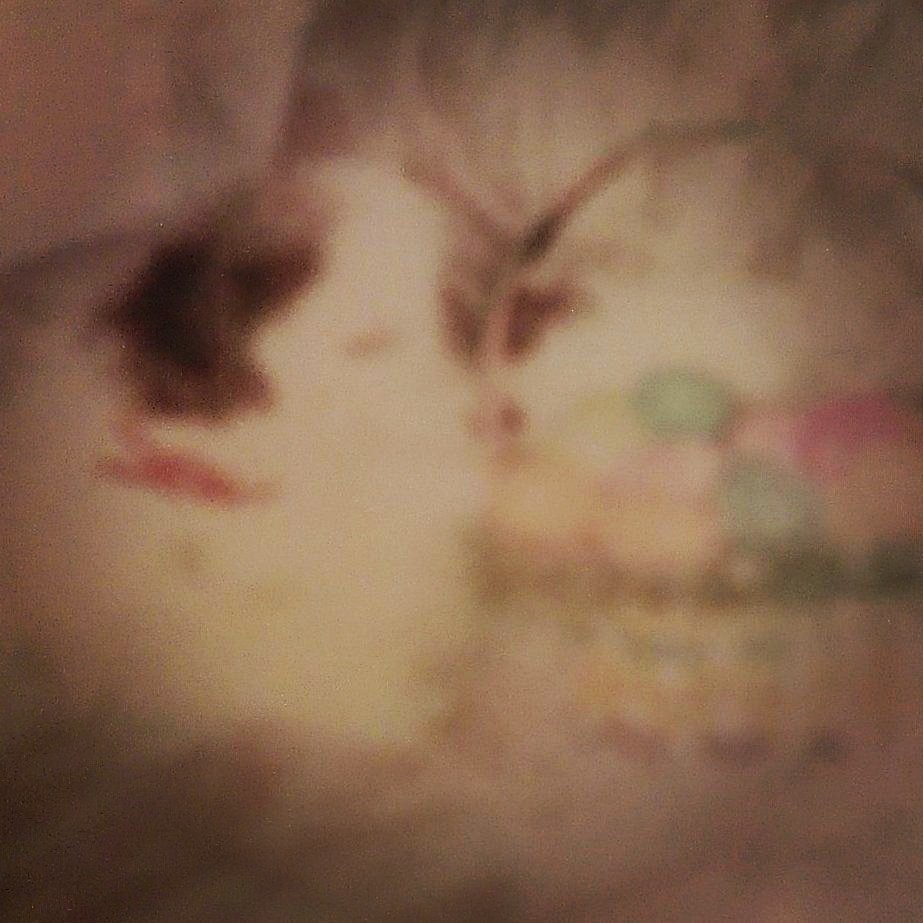The image is highly blurry and out of focus, primarily showcasing a brown background with a cream-colored center. The focal point appears to be a white dog with dark, hairy ears, a pointy snout, a black nose, and closed eyes, adorned with a red collar. The dog is positioned on the left side of the image, its head facing towards the right. On the right side of the image, a woven Easter basket is faintly visible. The basket's base features a lattice design with lateral bands in shades of purple, orange, and possibly green. The basket has a rim and an arched handle, and is filled with around ten brightly colored eggs at the top. The entire scene is indistinct, giving the appearance of a drawing or a screen.